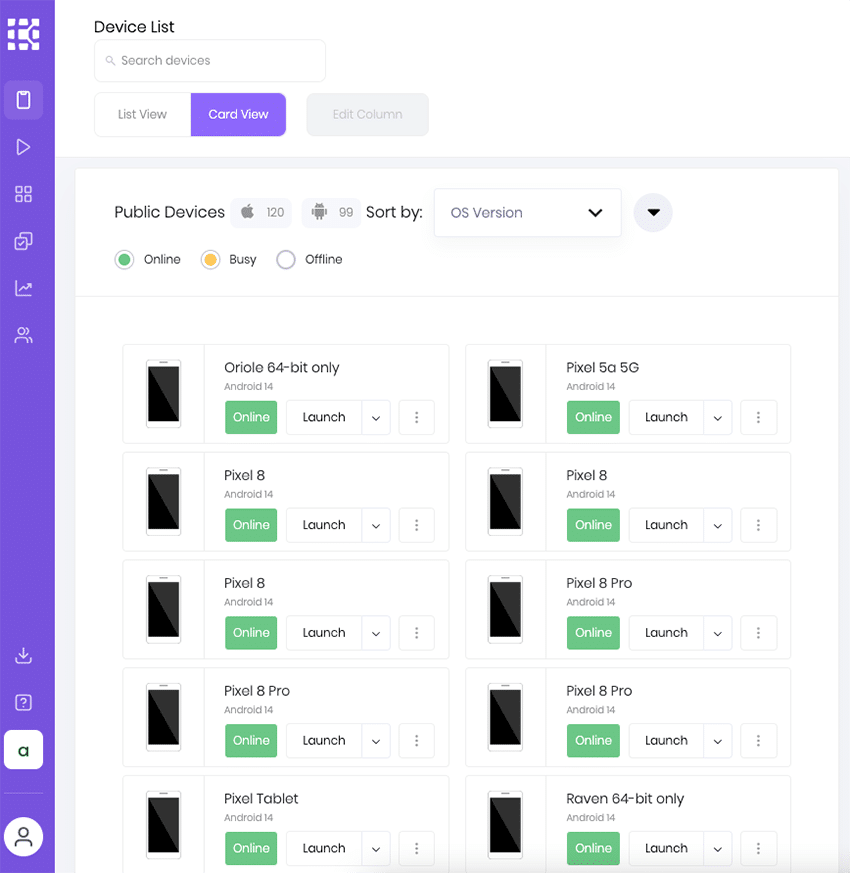This is a detailed photograph of an application or website interface showcasing various cell phone options. The background features a light gray color with a prominent white rectangle overlay and a white header. At the very top of the header, there is black text that reads "Device List." Directly below this header, there's a search bar with a gray magnifying glass icon and gray placeholder text that states "Search devices." 

Beneath the search bar, there are three buttons. The leftmost button is white with gray text that says "List View." Next to it on the right is a purple button with white text that says "Card View." Situated to the right of these two buttons is a standalone light gray button with grayed-out text that reads "Edit Column."

On the left side, there is a vertical purple sidebar, presenting a white logo composed of nine squares arranged in a grid. Below the logo, a series of icons are displayed vertically:
- A clipboard icon, which is currently highlighted,
- An arrow pointing to the right,
- A grid of four outlined squares,
- Two stacked squares with the front square featuring a checkmark,
- A line chart,
- An icon depicting a profile picture,
- A download icon,
- A question mark icon,
- A white square with rounded corners and a green "A" in the center.

Further down the sidebar, there's a thin white separating line, followed by a round white object featuring a black person icon.

In the main white portion of the page, there is a section labeled "Public Devices." To the right of this label, two light gray rectangles display logos: an Apple logo accompanied by the number "120" and an Android logo accompanied by the number "99."

The list of cell phones displayed under "Public Devices" includes the following models, each with a green "Online" button beneath the name and a white "Launch" button to the right:
- Oreo (64-bit only),
- Pixel 8,
- Pixel 8,
- Pixel 8 Pro,
- Pixel Tablet,
- Pixel 5a (5G),
- Pixel 8,
- Pixel 8 Pro,
- Pixel 8 Pro,
- Raven (64-bit only).